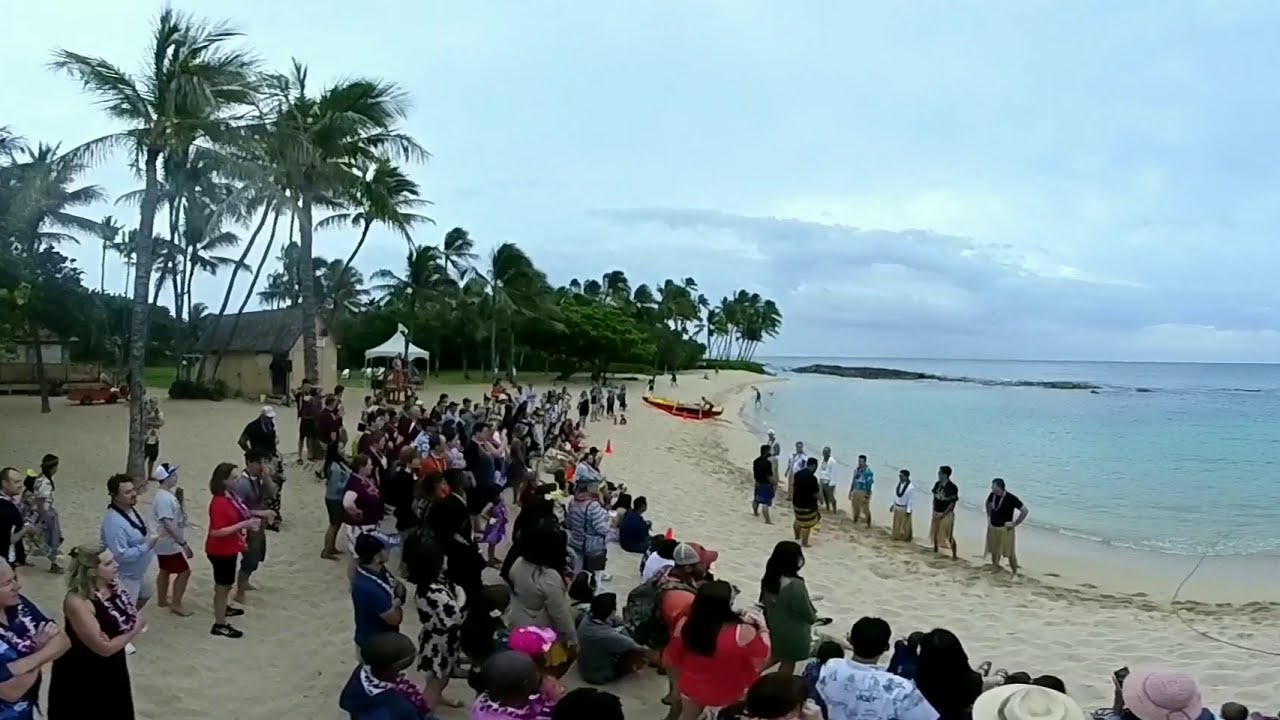In this captivating image, we're transported to a tropical beach, likely in a Hawaiian island setting where a hula or luau performance is taking place. A large, diverse crowd of tourists, ranging from 50 to 80 people, gather on the pristine, sandy shore to witness the performance. Many spectators are adorned with leis, contributing to the festive atmosphere. In the center, seven performers dressed in traditional grass skirts stand poised to begin a tribal dance. 

The backdrop features picture-perfect elements of island life with crystal clear blue waters gently lapping against the shore, and a cluster of palm trees and various tropical flora swaying under an overcast sky, hinting at the early evening or late afternoon. A beached canoe lies nearby, potentially brought in by a local, adding to the scenic coastal vibe. Huts, small tents, and a temporary white shelter can be seen in the distance, enhancing the authenticity of the tropical beach scene. This detailed snapshot captures the essence and vibrancy of an island celebration, beautifully framed by nature's tranquil grandeur.